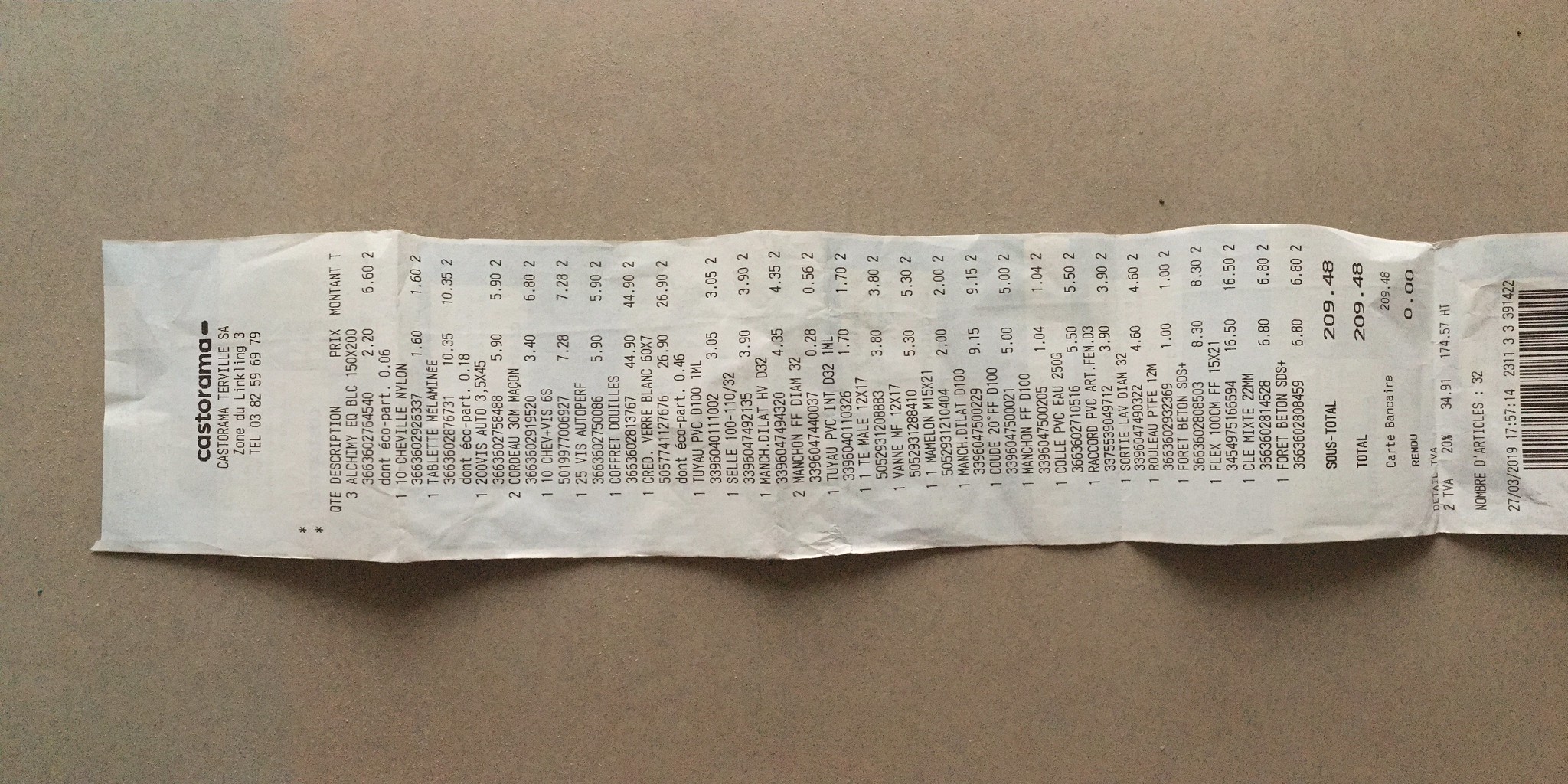An overhead photograph captures a horizontal receipt from Castorama, prominently displaying its logo in black lowercase letters at the top, followed by the store’s address. This exceptionally long receipt, filled with a multitude of listed items, extends from the image’s left to its right. A large rectangular barcode, partially cut off, appears towards the right center, indicating the end of the receipt. The entire document is set against a tan background, accentuating the creases where it had been previously folded – noticeable at the top, middle, and lower sections. The total expenditure, clearly printed as $209.48, highlights the extensive shopping reflected on this detailed and lengthy receipt.